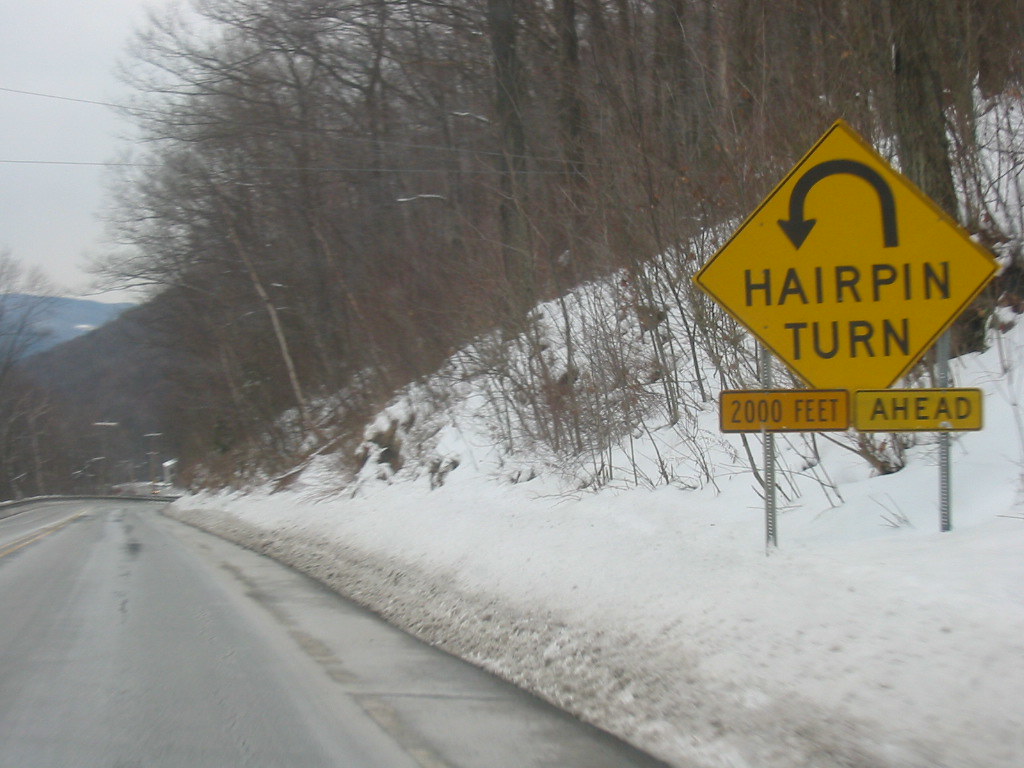A photograph taken on a cloudy winter day captures a two-lane road freshly plowed, with its double yellow stripe leading from the lower left corner across the image. To the right, the road swiftly rises into a small hill. In the foreground, a large yellow diamond-shaped sign with a curved arrow warns drivers of a hairpin turn 2,000 feet ahead. The overcast sky and barren winter landscape amplify the sense of caution projected by the road sign.